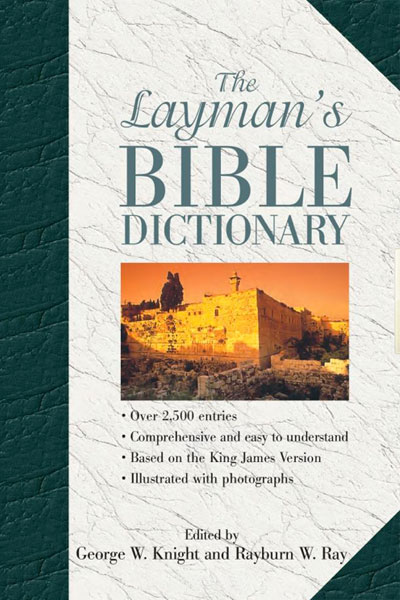The image depicts the cover of "The Layman's Bible Dictionary," edited by George W. Knight and Rayburn W. Ray. The multi-colored background features a mix of green, white, orange, yellow, black, and gray hues, characterized by a unique stone marbled theme. The dark green spine on the left side transitions into a gray stone texture across the rest of the cover, with matching green triangular accents in the top and bottom right corners.

Central to the cover is an image of an old, historic building, possibly biblical ruins, set against an orange sky. This building, appearing golden and somewhat crumbling, evokes a sense of ancient, religious significance, potentially from Jerusalem or a similarly historic site.

The text on the cover prominently states the title, "The Layman's Bible Dictionary," and provides key details: "Over 2,500 entries, comprehensive and easy to understand, based on the King James Version, illustrated with photographs." This text is organized with the title at the top and additional descriptions at the bottom, framing the central image.